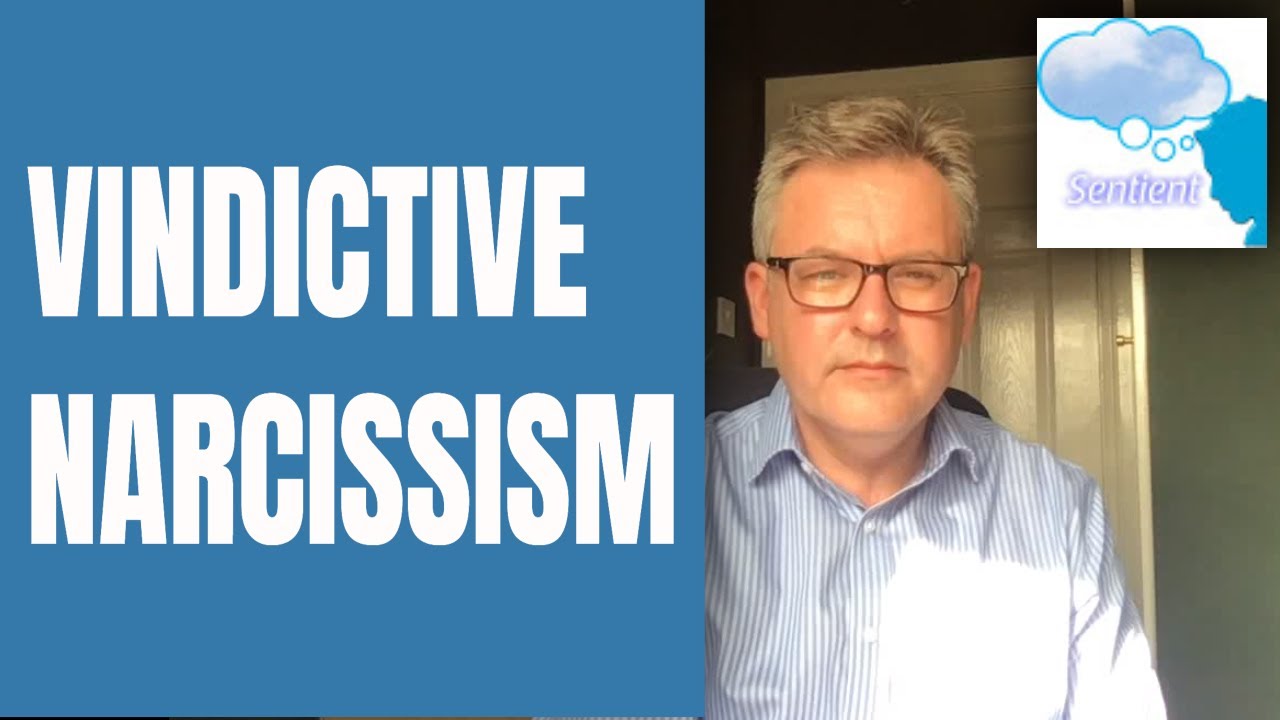This image integrates photographic realism with graphic design and typography, focusing on a middle-aged man and some textual elements. The image is primarily divided into two sections: on the left is a medium blue square with bold white text that reads "VINDICTIVE NARCISSISM" in all capital letters, spanning two lines. On the right side, there's a color photograph of a man with grayish light brown hair, dark eyeglasses, and a blue and white striped button-down long-sleeve shirt. He stands facing the camera with a neutral expression, against a background featuring a greenish-olive wall, a cream-colored door, and a light switch. In the top right corner of the image, there is a logo: a stylized profile of a person's head in dark blue with a blue-outlined speech bubble and the word "Sentient" beneath it. The predominant colors in the image are blue, white, peach, gray, and olive green. The overall presentation suggests it could be a part of an online meme or a presentation slide.